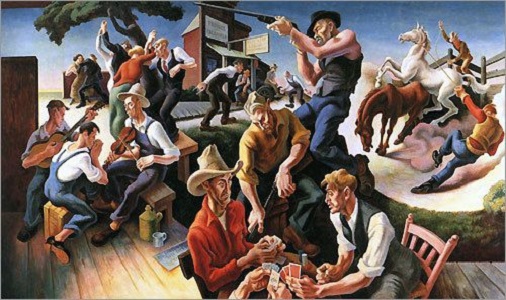In this detailed digital or hand-painted artwork, we see a dynamic scene of cowboys engaged in various activities, capturing the essence of a lively western celebration. Central to the image are a couple of people playing a game of poker, surrounded by others who partake in the festivities. To the right, two cowboys are attempting to wrangle a white and a brown horse, with one cowboy seemingly seated nearby with a lasso. The background reveals more cowboys, some playing musical instruments like a violin, tambourine, and guitar, while others appear to be dancing or potentially fighting. Overhead, a man is sighting down the barrel of a gun, adding an element of tension to the otherwise merry scene. Amidst this vibrant tableau, various shades of brown, tan, green, white, red, orange, blue, and silver can be seen, enriching the detailed environment. A small building with an unreadable banner frames the background, enhancing the scene's setting, which could easily be found hanging in a themed establishment.